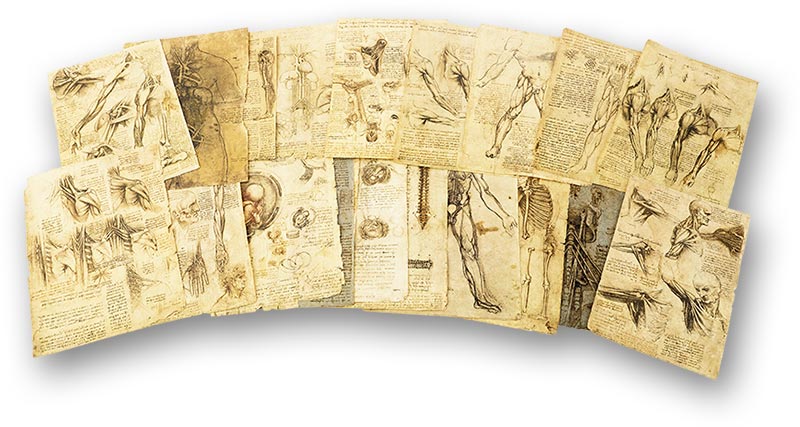The image captures an arch arrangement of 18 overlapping pages, meticulously detailed with intricate anatomical drawings and illustrations depicting various aspects of the human body. Among the illustrations are detailed depictions of muscles, veins, the skeletal system, including the spine and clavicles, and even prenatal images of a child. The pages resemble a collection from an antique medical journal or historical medical texts, giving off an aged appearance with weathered paper in hues of brown, cream, white, and black. Although the text on the pages is present, it is too small and faint to be legible, suggesting a fine use of technical language common in historical medical documentation. The overall presentation is clean, with a plain white, photoshopped background adding a subtle artificial shadow, keeping the focus entirely on the medical illustrations.